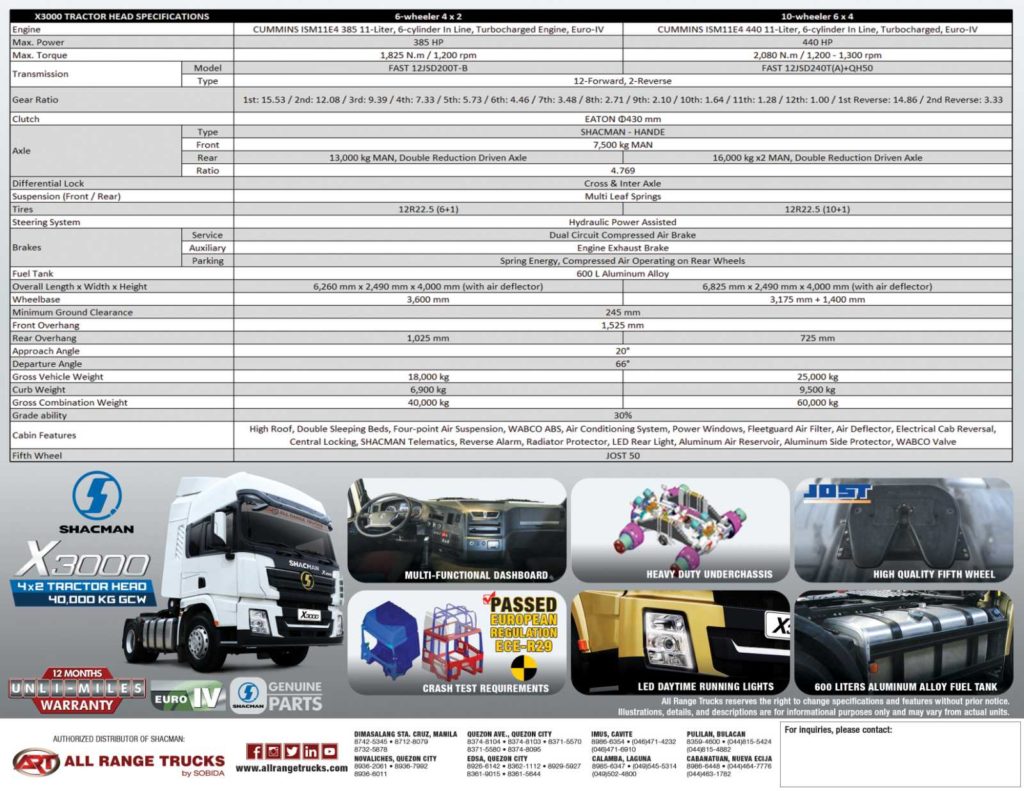The image is a detailed black-and-white product sheet from a company named Shackman, specializing in the transportation and parts industry. This product sheet is focused on the specifications for a tractor head, commonly used for 18-wheelers. The sheet includes an exhaustive inventory of auto parts and specifications such as fuel tank, engine, clutch, curb weight, grade ability, and cabin features.

In the middle section of the product sheet, there's a series of images highlighting key components and features of the tractor head. One image shows the interior dashboard, another displays the engine, which is noted as 'heavy duty under chassis.' There's also an image of the cabin, featuring LED daytime running lights and a high-quality fifth wheel. The sheet indicates that the bumper meets European crash test regulation requirements.

Additional images depict components such as a fuel tank and highlight features like the ability to lift 500 units. Underneath these images, the product sheet mentions 'all range trucks,' further emphasizing the versatile application of these truck parts.